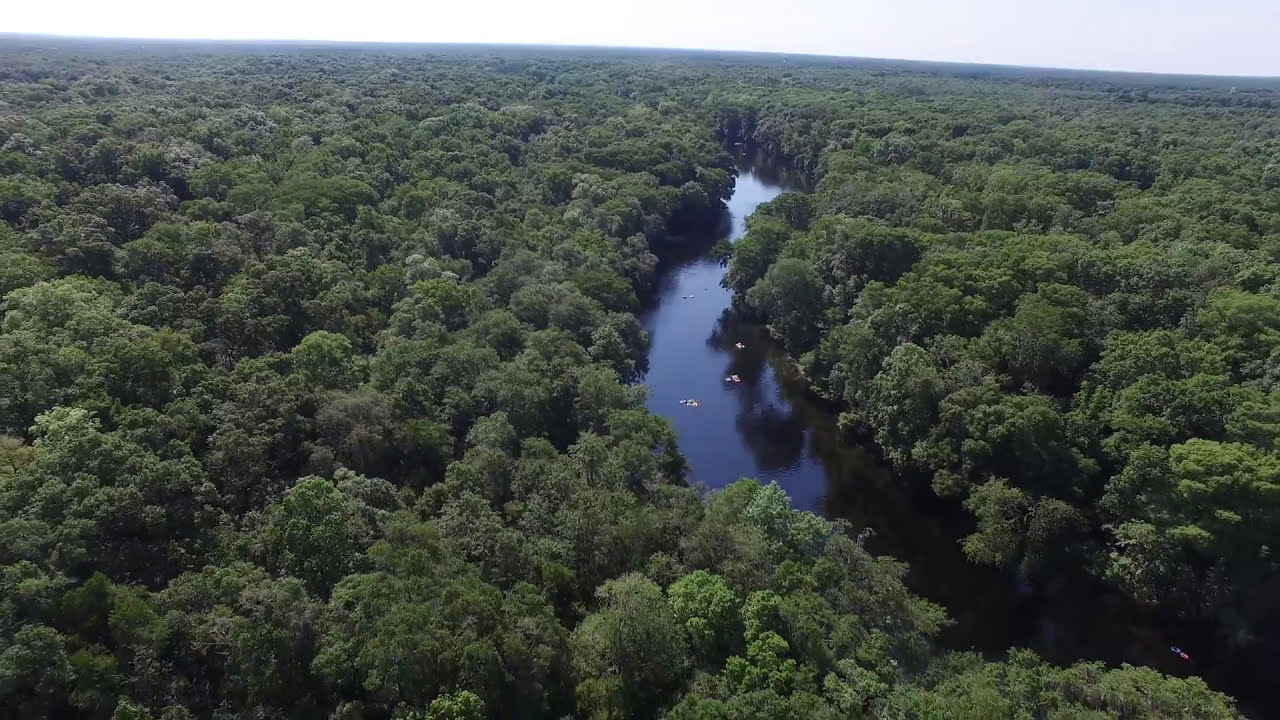This is an aerial view of a vast, flat forest landscape dominated by dense, lush greenery that stretches all the way to the horizon. A dark green river meanders through the center of the image, starting from the bottom right corner and winding its way upward and to the left, becoming partially obscured by the thick canopy of trees. The river, dotted with approximately five small boats concentrated in the middle and one in the bottom right, blends seamlessly into the surrounding verdant jungle. The overall scene exudes a sense of calm and untouched natural beauty, with no visible man-made structures disrupting the endless sea of green leaves. The photograph is slightly tilted, giving a unique, somewhat informal perspective, despite the stillness and tranquility of the setting. Above this serene landscape, the sky appears as a thin, dark gray band at the very top of the image, adding a dramatic contrast to the vibrant forest and river below.